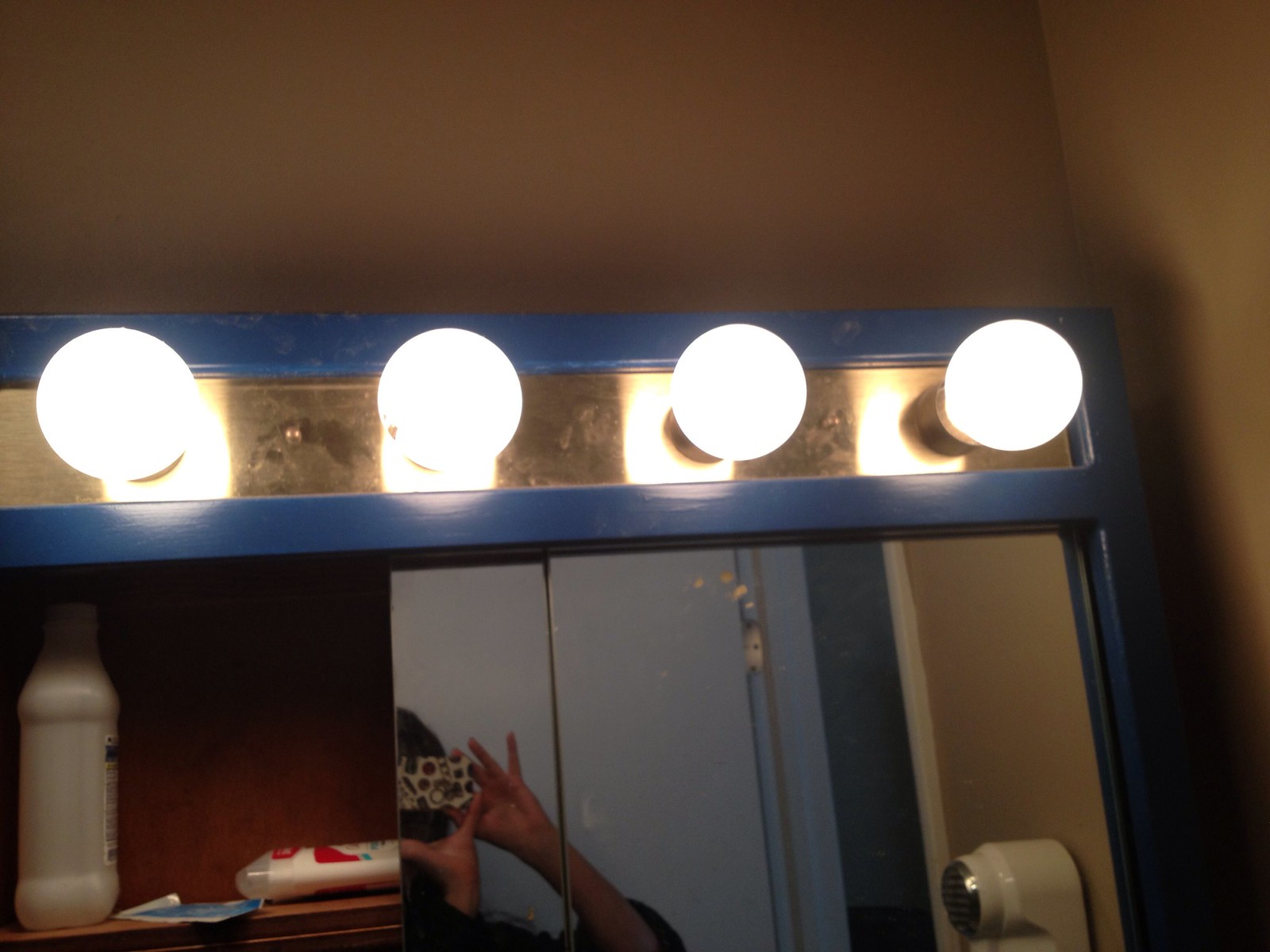This photograph captures the top section of a bathroom medicine cabinet. The wall in the background is brown, and atop the mirrored cabinet are four illuminated, Hollywood-style makeup lights. The mirror, framed in blue, partially reflects a person taking the picture with their phone, revealing only the top of their head, hands, and phone covered in a white case with colorful designs. The cabinet's mirrored door is slightly ajar, exposing contents inside, including a tube of deodorant lying on its side, a Q-tip, and a bottle that could be either mouthwash or rubbing alcohol. Additionally, a wall-mounted apparatus, possibly a blow dryer, is also visible in the reflection.